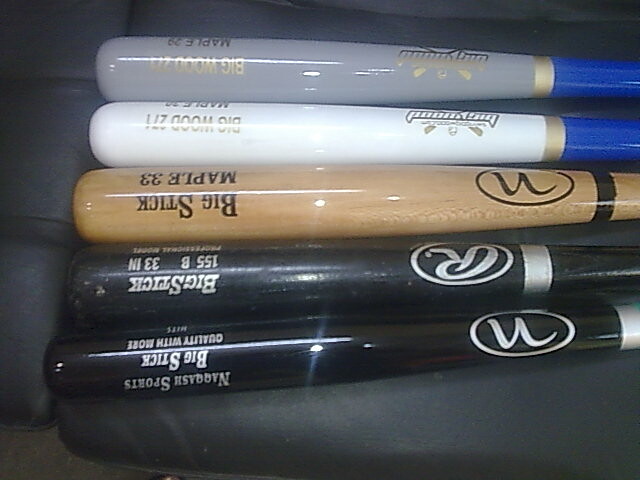The image depicts five baseball bats arranged horizontally against what appears to be a black or navy-blue cushioned surface, likely part of a couch. The bats are positioned with their handles pointing towards the right side of the image, though the very bottom of the handles is cut off from view. The bats display various colors and designs: the top one is light gray with a blue handle and a gold band near the handle, the second one is white with a similar blue handle and gold band, the middle bat has a natural wooden finish with black writing and a black band, and the bottom two are black with silver lettering and bands. All bats have writing that appears upside down, making it challenging to fully decipher the text, though the word "Rawlings" and the phrase "Big Stick" can be partially identified.